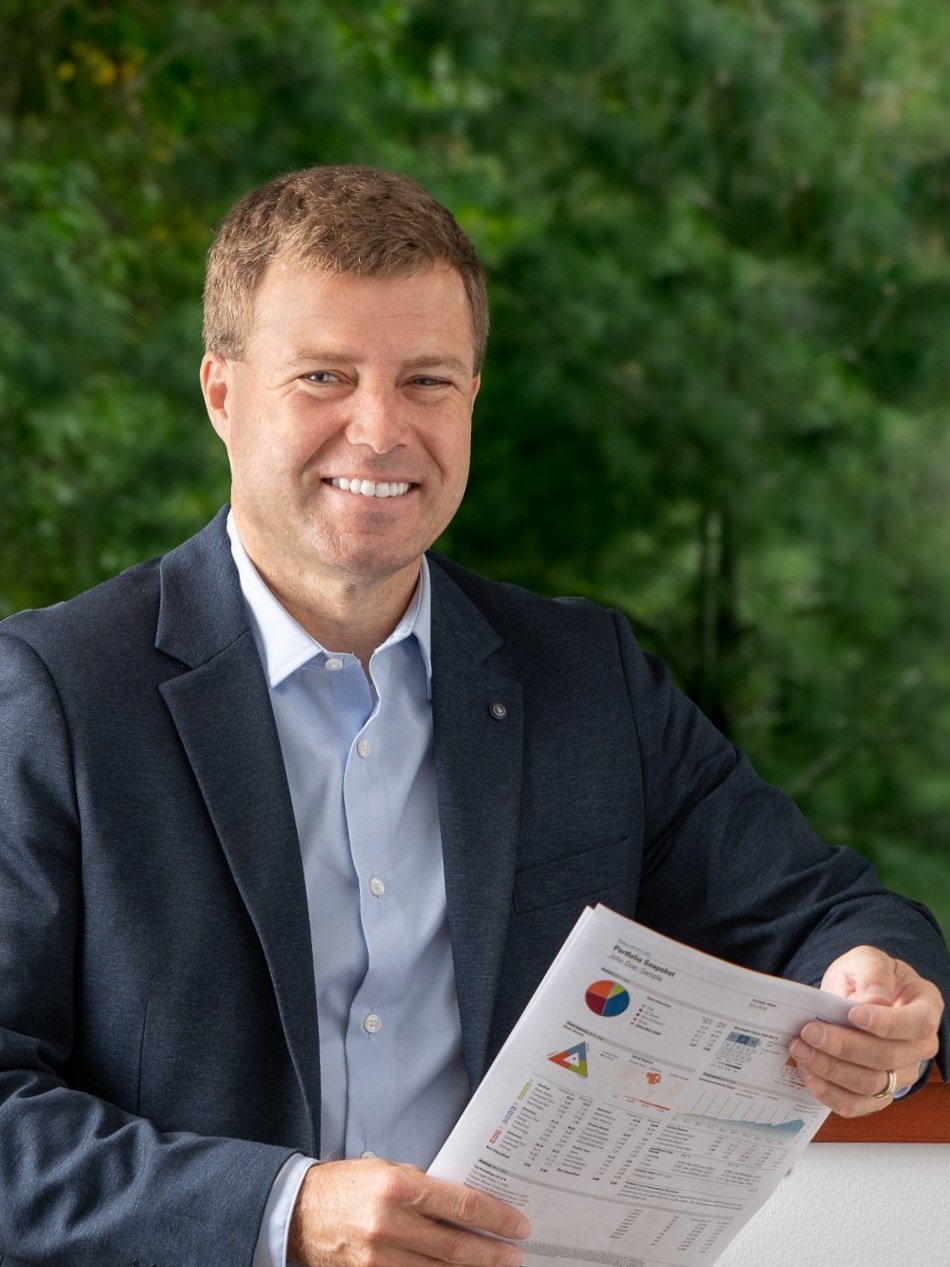This photograph features a Caucasian man with short light brown hair and neatly trimmed nails, dressed in a navy suit jacket over a light blue collared shirt, sans tie. He is wearing a gold wedding band on his left hand. The background is slightly blurred, featuring foliage and trees, suggesting the photo was taken outdoors during the day. The man, who exudes financial stability and well-being, is smiling warmly at the camera, his eyes crinkled in a genuine smile. He holds a portfolio snapshot filled with various graphs, charts—some in colors like orange, green, blue, and red—and lists. The document, marked with the title "John Doe Sample," suggests this may be an advertisement or stock photo illustrating financial prosperity and competence.